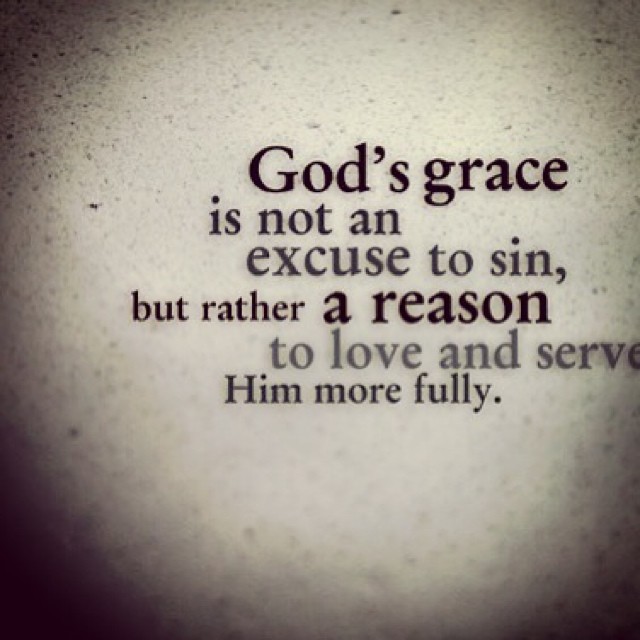The image displays a textured, speckled gray background with a spotlight effect that darkens towards the corners. In the center-right of the image, the text reads: "God's grace is not an excuse to sin, but rather a reason to love and serve Him more fully." The text varies in color from black to different shades of gray and is presented in different sizes, with "God's grace" and "reason" being notably larger for emphasis. The overall image is clear and easy to read despite some graininess in the background.